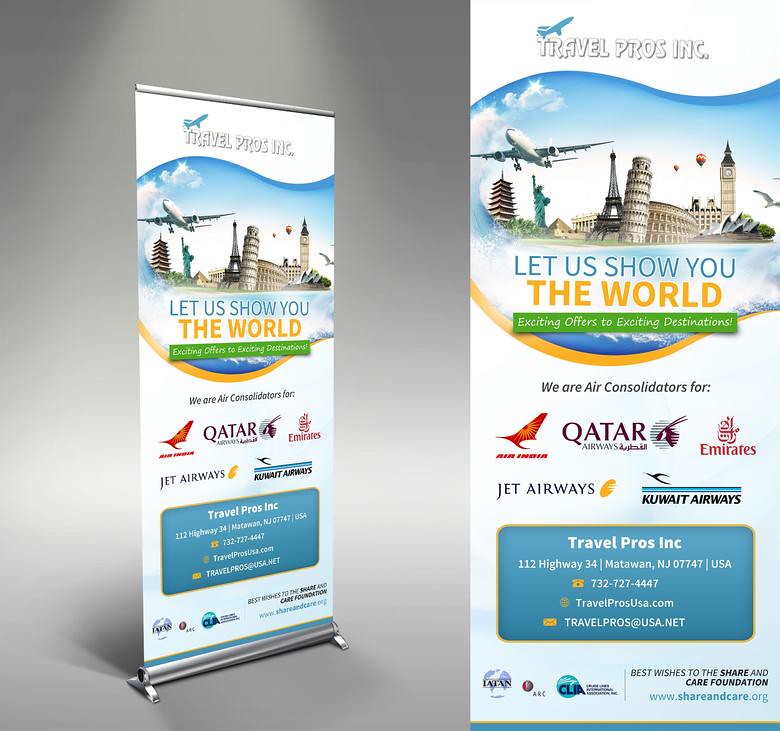The image depicts a standing banner supported by two pegs and a metal rod, positioned against a gray background. The banner, promoting Travel Pros, Inc., is richly detailed with various vibrant colors including gray, white, blue, green, red, orange, purple, yellow, and light blue. The top portion showcases a blue airplane taking off, flying over a montage of iconic landmarks such as the Eiffel Tower, Leaning Tower of Pisa, Colosseum in Rome, Big Ben in London, the Statue of Liberty, the Capitol building in Washington D.C., and a recognizable Japanese structure. Additional elements like seagulls and famous buildings contribute to the travel-themed design. The text on the banner reads: "Travel Pros, Inc. Let us show you the world. Exciting offers to exciting destinations." It highlights their role as air consolidators for airlines including Air India, Qatar Airways, Emirates, Jet Airways, and Kuwait Airways. The banner also provides the company's address—112 Highway 34, Matawan, NJ 07747, USA—and contact information, featuring a phone number, (732) 727-4447, and a website, TravelProsUSA.com, along with an email, TravelProsAtUSA.net. The right side of the image shows a zoomed-in section of the banner, emphasizing the detailed advertisement for the travel agency.